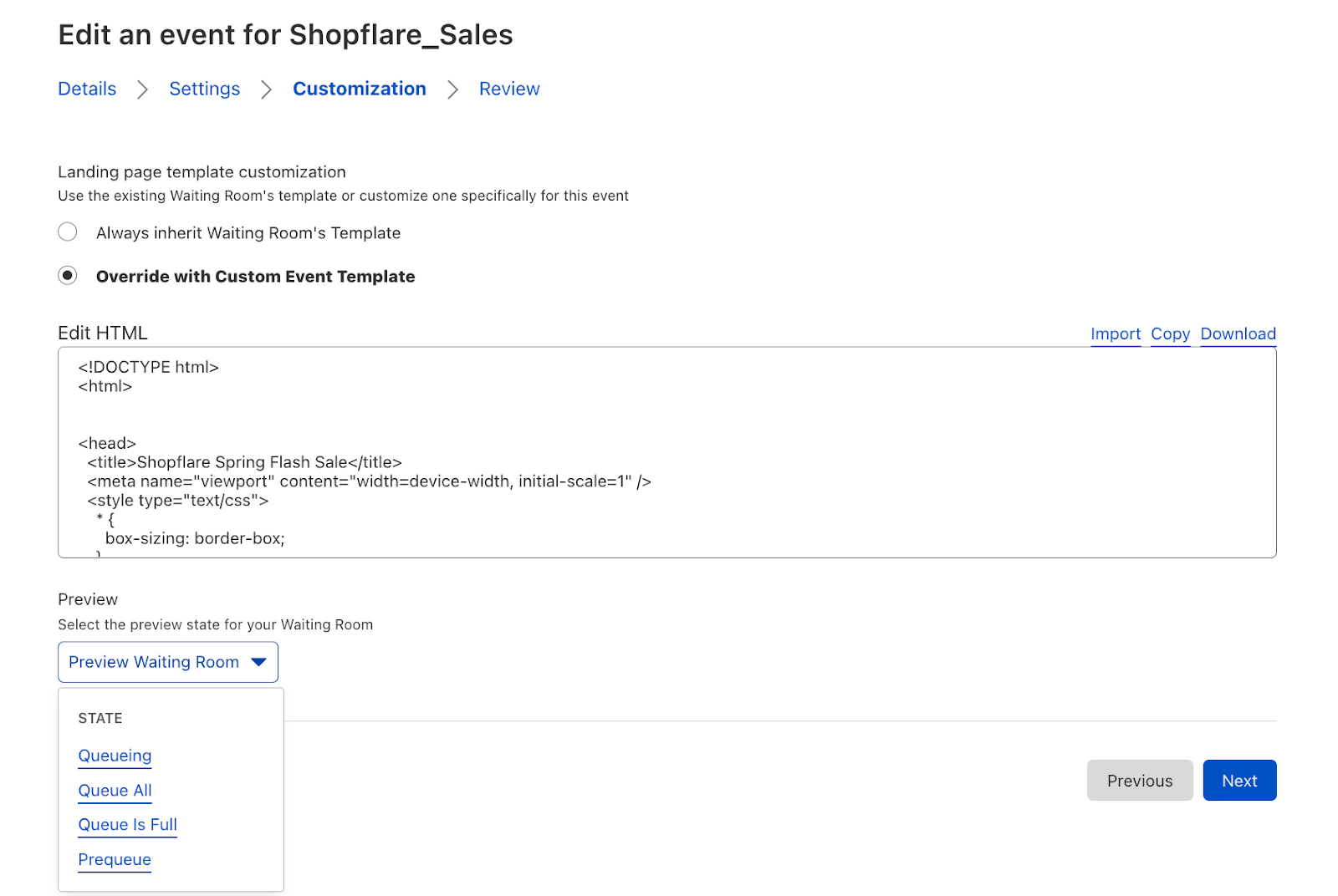Screenshot of the event editing interface for "shopflare_sales" with a comprehensive breakdown of customization options.

In the upper left corner, the title "Edit an Event for shopflare_sales" is displayed. Below the title, there is a navigation line with tab options: "Details," "Settings," "Customization" (highlighted), and "Review," each marked with a caret pointing to the right.

The main section shows "Landing Page Template Customization," guiding users to either use the "existing waiting rooms template" or "customize one specifically for this event." Two radial buttons are presented as choices: the first one, labeled "Always Inherit Waiting Rooms Template," and the second one, labeled in bold black letters "Override with Custom Event Template," which is selected with a black dot inside the white circle.

Below these options is a long rectangular text box for editing HTML, prefaced by the text "Edit HTML." The box displays sample markup starting with "<!DOCTYPE html>." Functions to "Import," "Copy," and "Download" are available in blue links at the top right of this box.

At the bottom, there is a "Preview" section urging users to "Select the preview state for your waiting room." It includes a dropdown menu labeled "Preview Waiting Room," offering four states: "Queuing," "Queue All," "Queue is Full," and "Pre-Queue."

On the right side of the interface, gray and blue tabs provide navigation, labeled "Previous" and "Next" respectively.